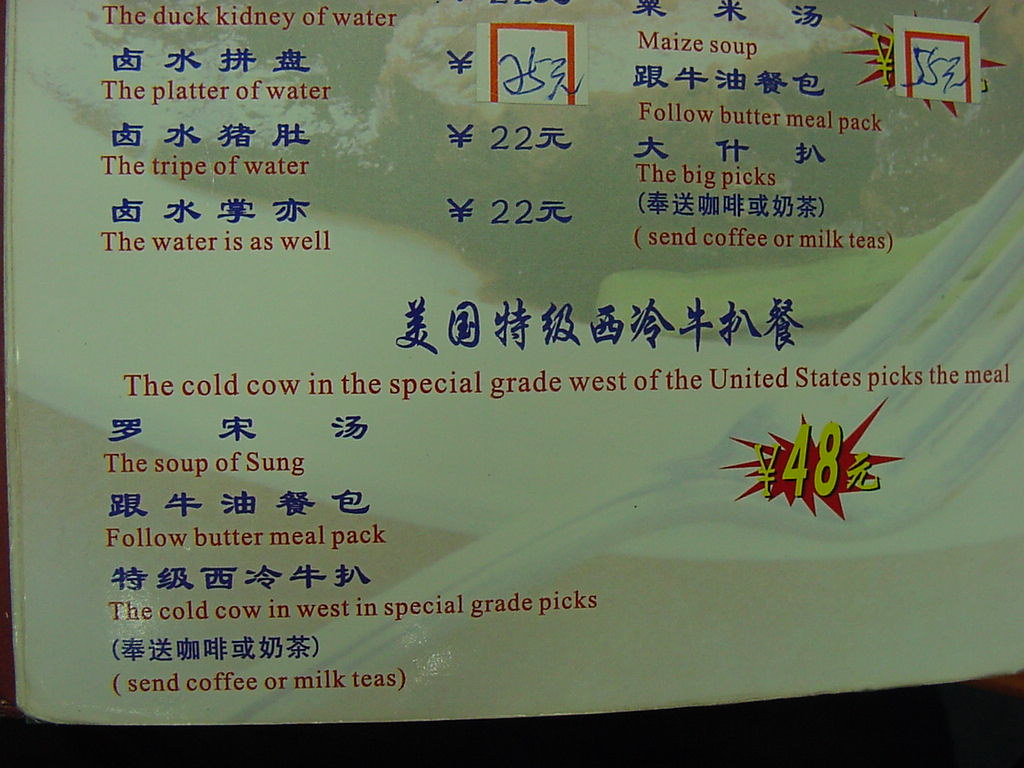This image depicts a bilingual menu featuring both English and Japanese or Chinese text. The menu displays a white background with a subtle watermark, likely illustrating a fork and a steak on a platter. The English text on the menu is prominently printed in red, while the Asian script appears in blue. Some notable, albeit quirky, menu items include phrases like "the duck kidney of water," "follow buttermilk pack," "send coffee or milk to the big pigs," and "the cold cow in the special grade west of the United States picks the meal." These peculiar translations suggest that the menu may be from a restaurant offering a diverse range of dishes with whimsical descriptions. The primary colors used in the design are white, red, and blue, enhancing its visual appeal and readability.